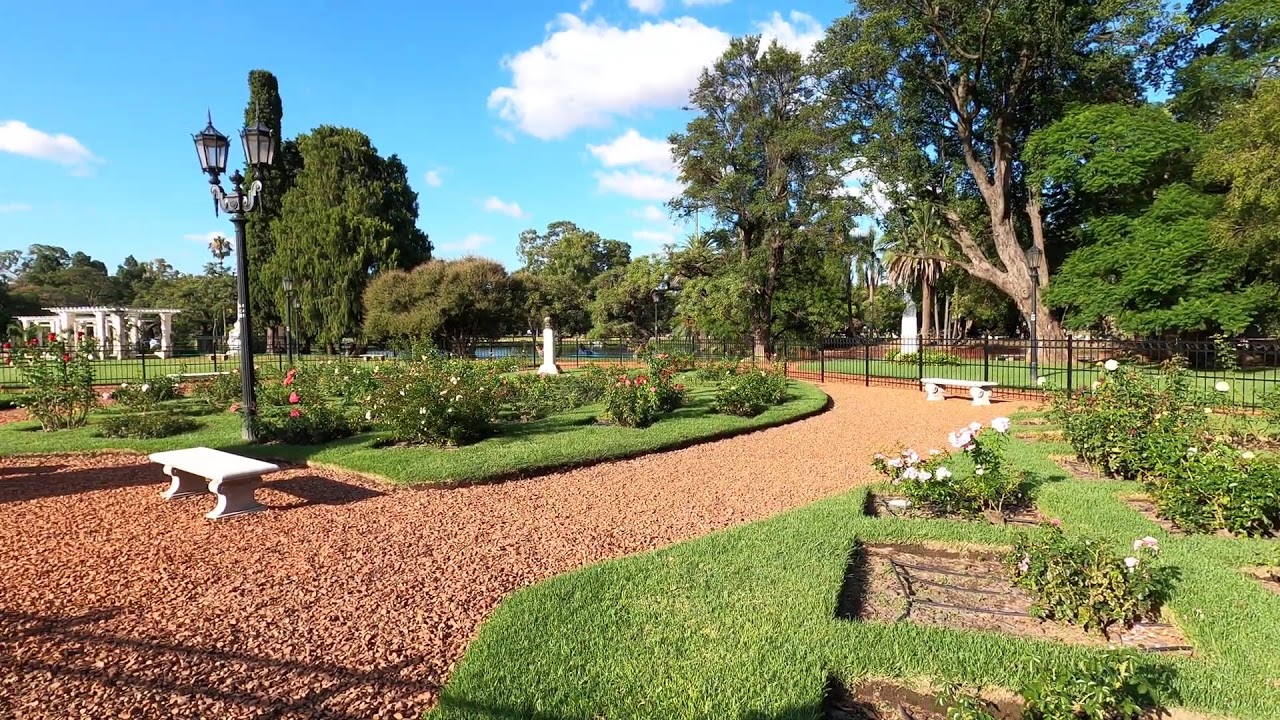This detailed photograph captures the serene beauty of an outdoor garden, which could be located in a public park or a private estate. The centerpiece of the garden is a well-maintained walking path made of brown-colored pebbles or mulch, leading into the tranquil setting. Along the path, there are small white benches inviting visitors to sit and soak in the surroundings. 

The garden is lush with meticulously cut green grass and an abundance of flowering plants, prominently featuring white and red roses that add a burst of color. There are also rectangular flower beds that seamlessly blend with the grass, creating an almost artistic patchwork pattern.

In the background, a variety of trees, including weeping willows and possibly mimosa trees, stand tall behind a classic black metal fence with posts. These trees contribute to the peaceful ambiance, complemented by elegant black lampposts with globe-shaped lights. The sun illuminates the scene under a bright blue sky adorned with a few white clouds, casting a warm glow over the entire landscape.

Further in the distance, a tranquil body of water, likely a small pond or lake, adds to the garden's picturesque charm. Additionally, a gazebo can be seen far off in the background, offering another spot for quiet reflection. Overall, this image captures a perfect daytime moment in a beautifully landscaped garden.